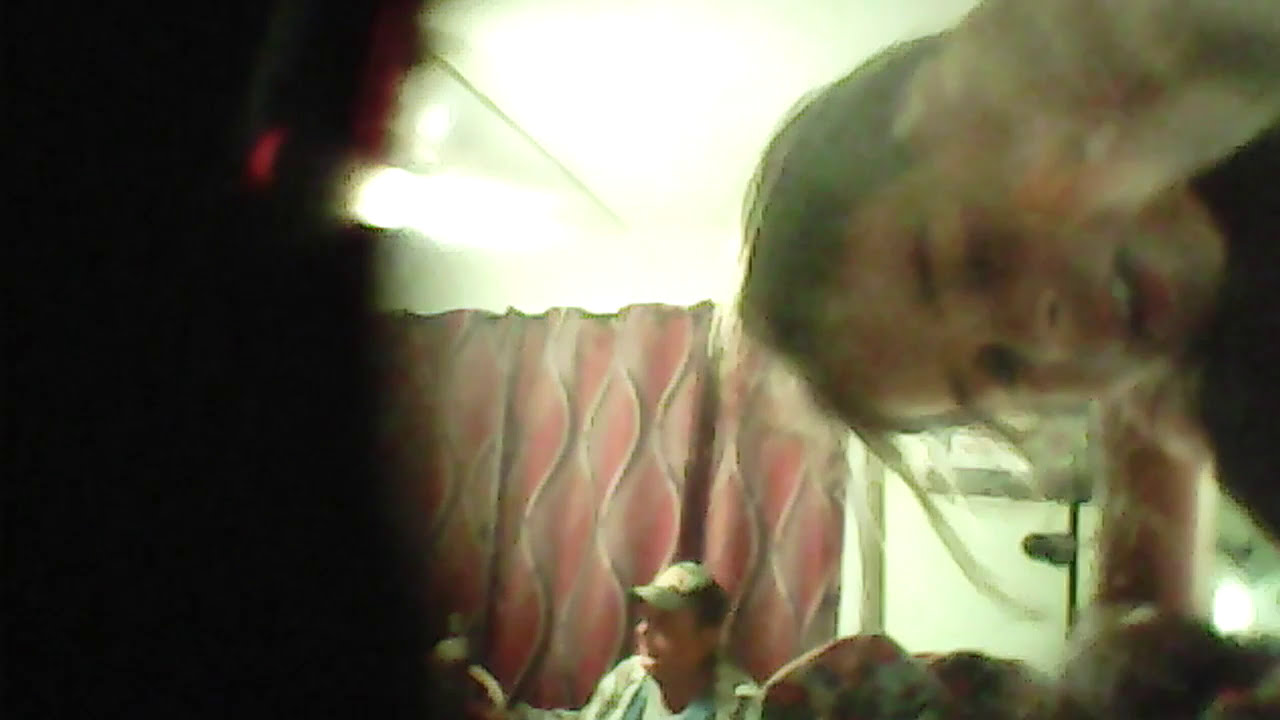The image depicts a very out-of-focus scene centered around a man seated near the bottom, wearing a light green hat and a multi-colored, long-sleeved, striped shirt in shades of blue, white, black, and brown. This man has a light-skinned complexion and his head is turned towards the left. Behind him is a maroon-colored curtain adorned with black, swirly lines that stretch vertically from the top to the bottom of the image. The upper part of the photo is washed out with light, possibly due to glare. On the right side, there's a young girl with brown hair, some strands hanging down, who is partially obscured by her own hand held up close to her face. She is light-skinned, her mouth slightly open, revealing her top teeth, and her brown eyelashes are visible, although her eyes are indistinct due to the blurriness. The left side of the image is obscured by a dark blotch or shadow, making it unclear. The overall setting includes some greenish and reddish hues, suggesting a dimly lit environment or possibly an artsy filter effect. The entire photograph has a hazy and unclear quality, making it difficult to discern finer details.